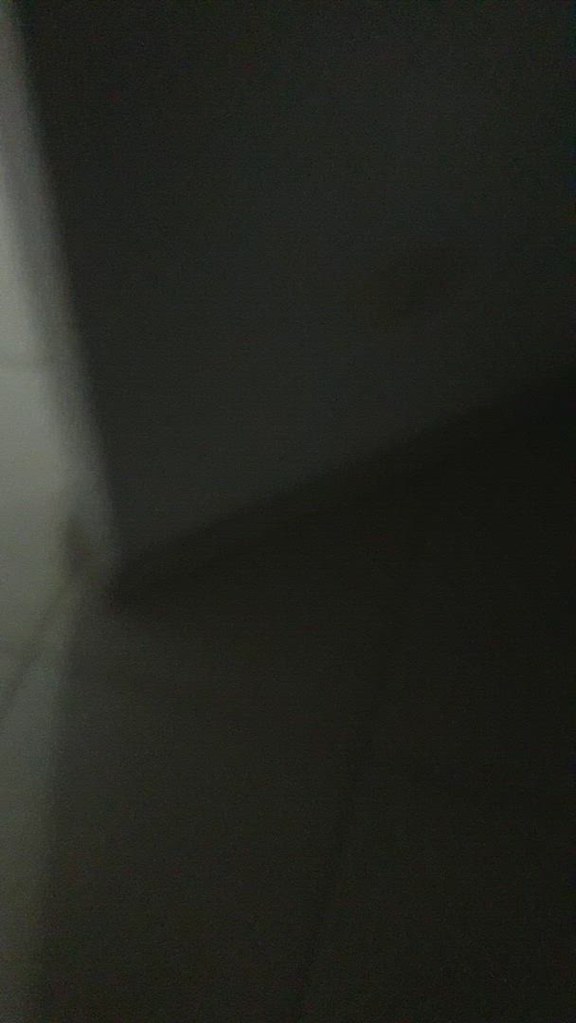This image depicts a dimly lit corner of a room, dominated by a pitch-black atmosphere. The focal point is the left corner, where a white wall meets the floor. The bottom of the image shows a whitish color gradually darkening towards the bottom right. A shadowy circle and a plank mounted on the bottom of the wall, which is brown, are also visible. The room's floor consists of large, square tiles with horizontal and vertical lines, and the tiles seem to be white but are obscured by dark shadows. The overall image is fuzzy, with a blurred, gray floorboard and indistinct, possibly gray elements in the deeper background. A few white lights can also be seen near the corner, contributing to the minimal illumination in the image.